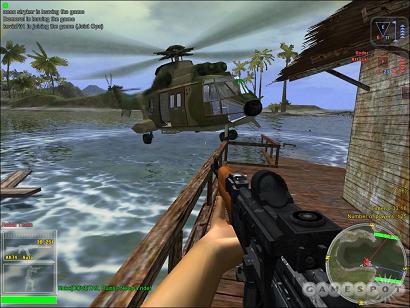A still from a video game showcases a person standing on a dock, holding a gun, as indicated by the first-person perspective. In the top left corner, there is some text that is too small to read. The dock, which features a brick building with a wooden roof, extends into the water. A helicopter is seen flying extremely close to the dock, while another helicopter is visible in the distance. The backdrop includes a beach lined with palm trees and mountains. The sky is overcast, casting a gray hue but without any rainfall. The watermark "GameSpot" is visible at the bottom of the image.